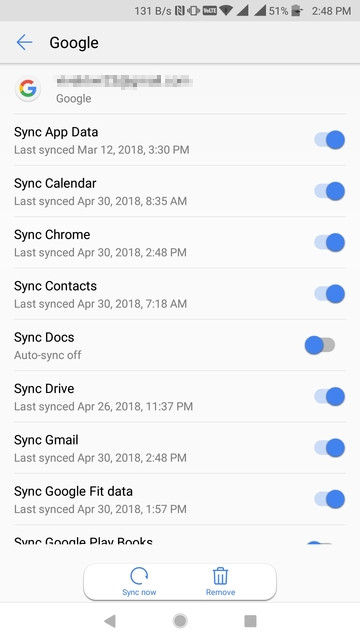The image depicts a screenshot from a cell phone showing a settings menu for Google. At the top of the image, the status bar is visible, displaying typical information such as the battery meter, Wi-Fi signal, clock, and other standard icons. Below the status bar, there is a header labeled "Google" accompanied by a back-arrow icon.

Directly beneath this header, the Google logo is prominently displayed. Following downwards, there are multiple settings options listed, each prefixed with the word "sync": "Sync app data," "Sync calendar," "Sync Chrome," "Sync contacts," "Sync docs," "Sync drive," "Sync Gmail," "Sync Google Fit data," and "Sync Google Play Books." Toward the bottom of the screen, there are additional interactive options labeled "Sync now" and "Remove," indicating actions the user can take. The overall layout and design are indicative of a standard Google account settings interface on a mobile device.